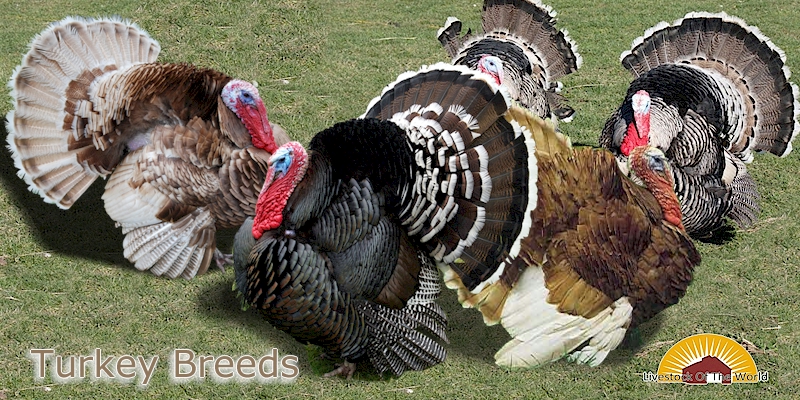The image is a digitally edited photograph of five turkeys, each representing different breeds, positioned on a vibrant green grassy field. The leftmost turkey showcases a mix of brown with white speckles and a distinct red head. Beside it, a turkey displays black plumage with brown and white tail feathers, also featuring a red head. Behind them, another turkey stands prominently with striking black and white feathers, accented by a red head and blue facial features. The center turkey, uniquely eye-catching, is predominantly black with an intricate design of black and white striped tail feathers, along with a brown fan trimmed with black and white edges. Another turkey exhibits a chocolate brown body contrasting with white feathers below. The turkeys all possess plump, rounded bodies with thick feathers, and their distinctive galls and vividly colored red heads are notable features. In the bottom left corner, brown text with a white border labels the image as "turkey breeds." The bottom right corner features a logo of a red barn with a sunburst behind it, accompanied by black text that reads "livestock of the world."